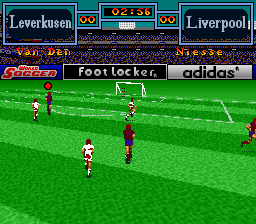The image showcases a vibrant, colorful scene from a computer soccer game. The meticulously detailed green field features alternating light and dark green stripes, created by mowing the grass in opposite directions. Miniature player figures are scattered across the field, with one team dressed in whitish uniforms and the opposing team in blue and red attire. In the backdrop, beyond the field, are the start of the stands, adorned with advertising banners. One black banner prominently displays "Foot Locker" in white lettering, while another white banner bears the "Adidas" logo in black letters. Above the field, the scoreboard indicates a match between Liverpool and Leverkusen, with the score currently tied at 0-0 and 2 minutes and 56 seconds remaining in the quarter.